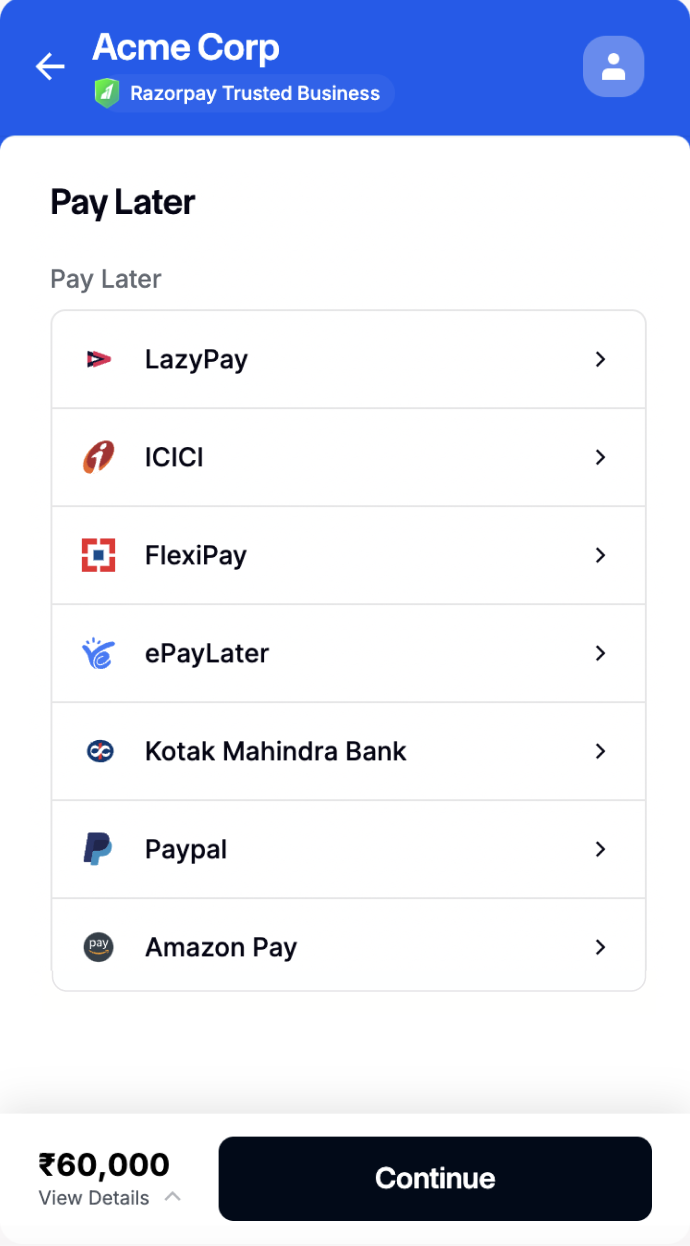The image is a screenshot of the Acme Corp interface. The top section features a horizontal blue bar stretching from left to right. On the left side of this bar, there is a small gap followed by a square icon with a lighter blue outline and a slightly lighter blue interior, showcasing a white, capitalized 'A' in its center. To the right of this icon, after another small space, the text "Acme Corp" is displayed. Below "Acme Corp," the phrase "Razorpay Trusted Business" is written in a smaller font. At the far right of the blue bar, there is a white 'X' icon, indicating the option to close the interface.

Beneath the blue bar, the screen transitions to a white background, prominently displaying the prompt "Select an option." Below this prompt, a list of payment options is featured sequentially: "Simple SIMPL," "LazyPay," "ICICI Bank Payletter," and "FlexiPay by HDFC Bank." Each option is presented as a separate clickable or selectable element.